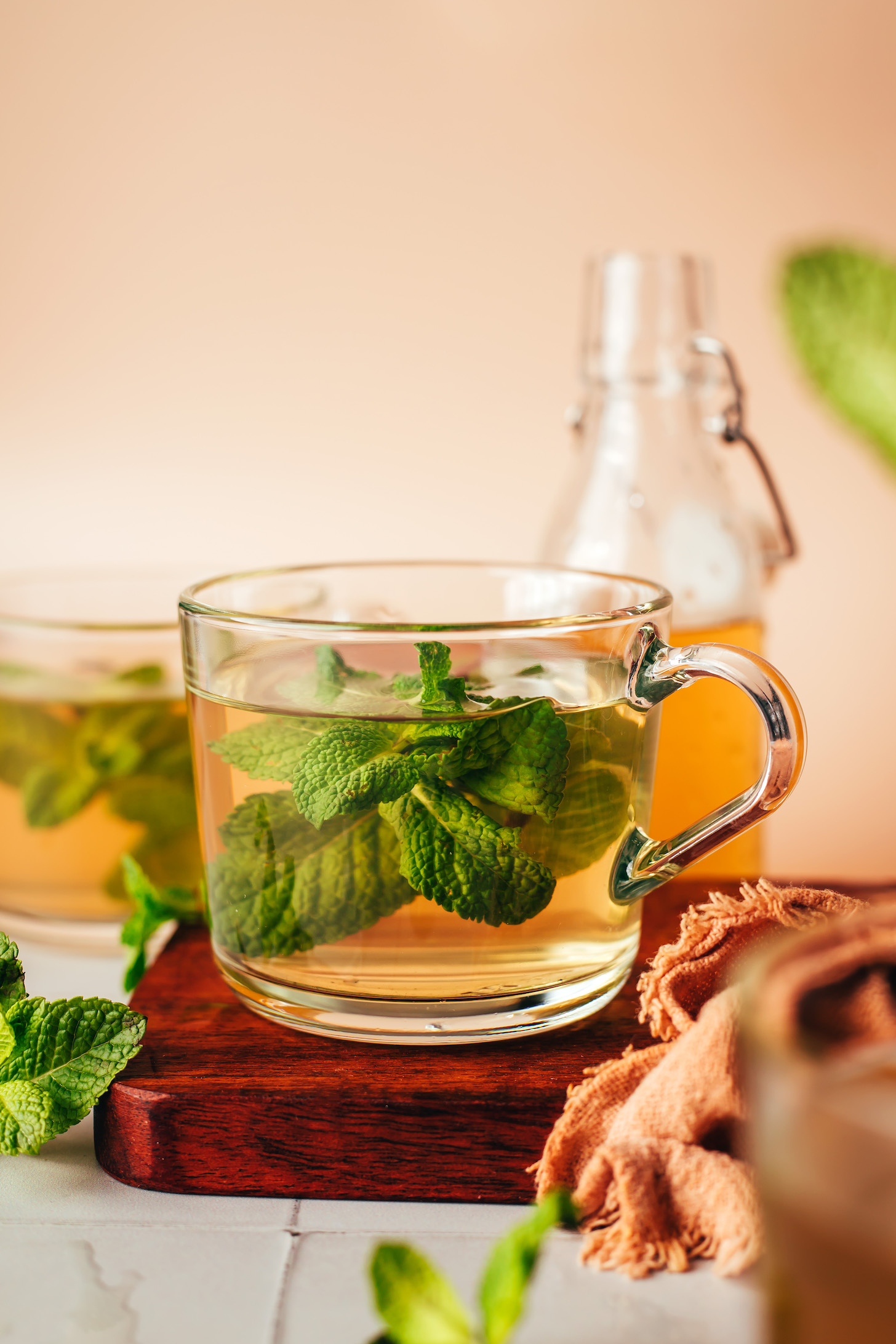This high-definition close-up photograph features a detailed arrangement centered around a brown, dark-stained wooden board. On this board, a clear glass mug is filled with a light yellow liquid, likely beer, that has fresh mint sprigs floating in it. To the right of the mug, an orange cloth, possibly a rag, extends over the edge of the board onto a marble white tile surface. Surrounding the board on the tile surface are additional sprigs of fresh mint. In the background, there is a second identical mug containing the same liquid and mint, emphasizing the consistency of the setup. Further back, a clear glass bottle with the same yellow liquid is visible on a peach-toned backdrop. The bottle features a cork lid that is fastened with metal, which is currently detached and hanging off the side. The overall composition and quality of the photo highlight the textures and colors in a vivid, eye-catching manner.